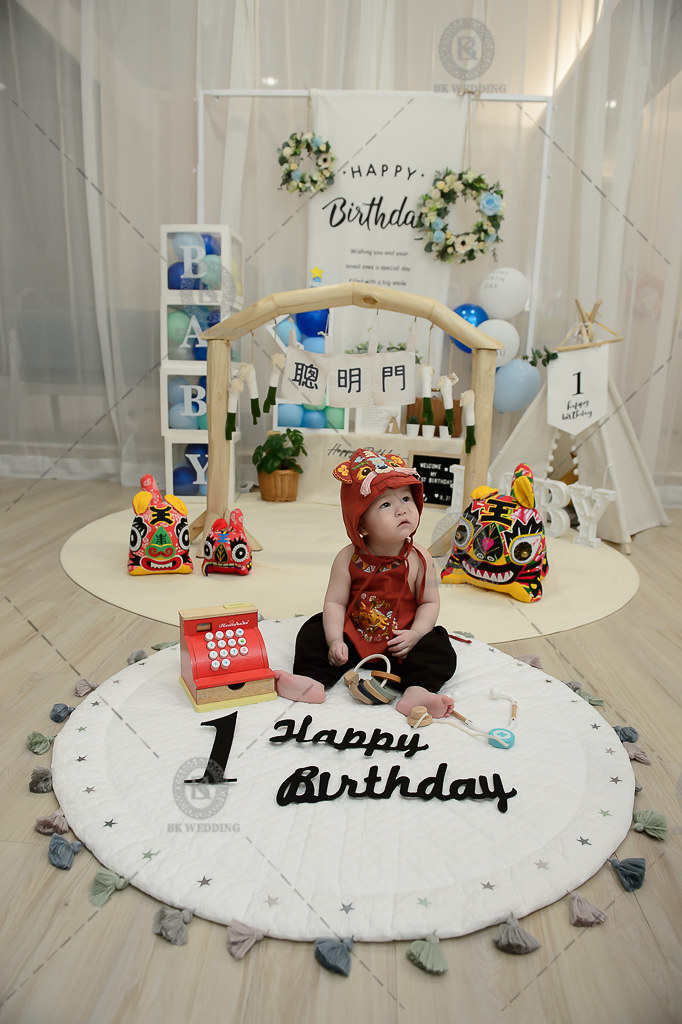The photograph depicts an indoor photoshoot celebrating an Asian baby's first birthday. The setting features a light-colored hardwood floor with two circular rugs: one in the foreground, with white, light gray, green, and pink tassels, and another behind it in a yellowish tone. Positioned centrally on the foreground rug, the baby is dressed in a red panda hat, a matching smock, and black pants. The baby sits near a toy cash register and various rattles. Surrounding the scene are meticulous decorations: a bamboo archway behind the baby holding three plush dragon characters and flanked by a white teepee on the right. On the left, four white crates spell out "B-A-B-Y" and each crate contains blue, light blue, and green balloons. A sheer white curtain and a squared archway frame the wall behind, adorned with a banner that reads "Happy Birthday" and two wreaths with green, light blue, and white flowers. The image is vibrant, showcasing colors such as tan, blue, green, purple, pink, white, black, and red, and captures the joyous atmosphere of the celebration.